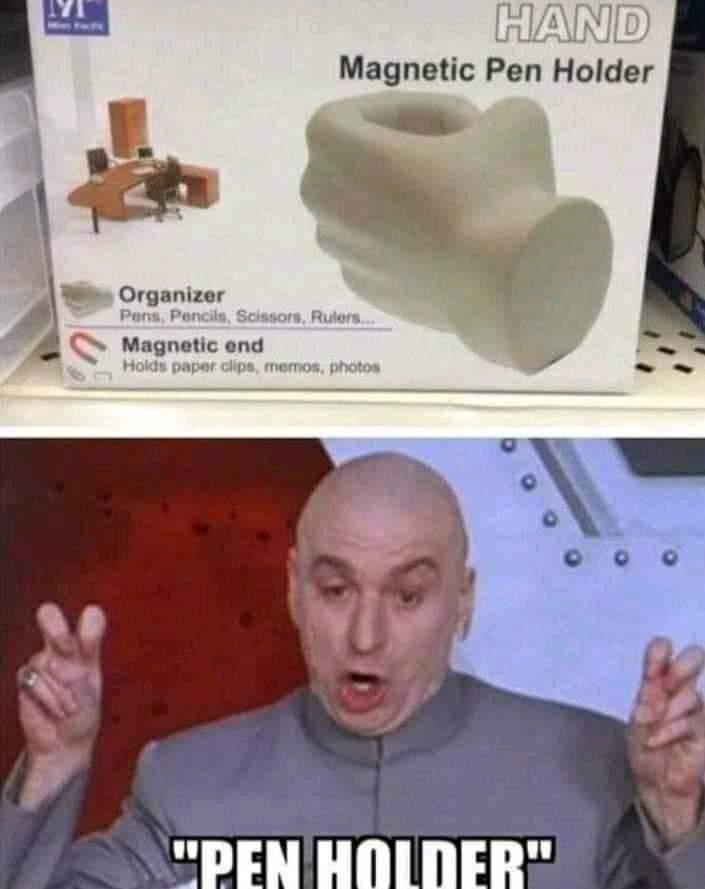The vertically aligned rectangular image features two distinct sections. The top part displays a package resting on a white metal shelf. The package is labeled "Hand Magnetic Pen Holder" and includes an illustration of a decorative hand making an open circle, designed to hold various office supplies like pens, pencils, scissors, and rulers. Additional text on the package highlights its "Magnetic End" that can hold paperclips, memos, and photos. In the bottom left corner of the package image, there's a subtle depiction of a desk with a computer. 

Below the product image is a meme featuring Mike Myers as Dr. Evil from Austin Powers. Dr. Evil, recognizable by his bald head and gray long-sleeved outfit, is shown making air quotes with both hands. His mouth forms an "O" shape, and his eyebrows are raised in a mocking expression. The bottom of this meme image is captioned with the words "PEN HOLDER" in all caps, white letters outlined in black, emphasizing the satirical tone. The overall color palette includes shades of white, gray, black, blue, and peach, contributing to the office setting and the humor of the meme.